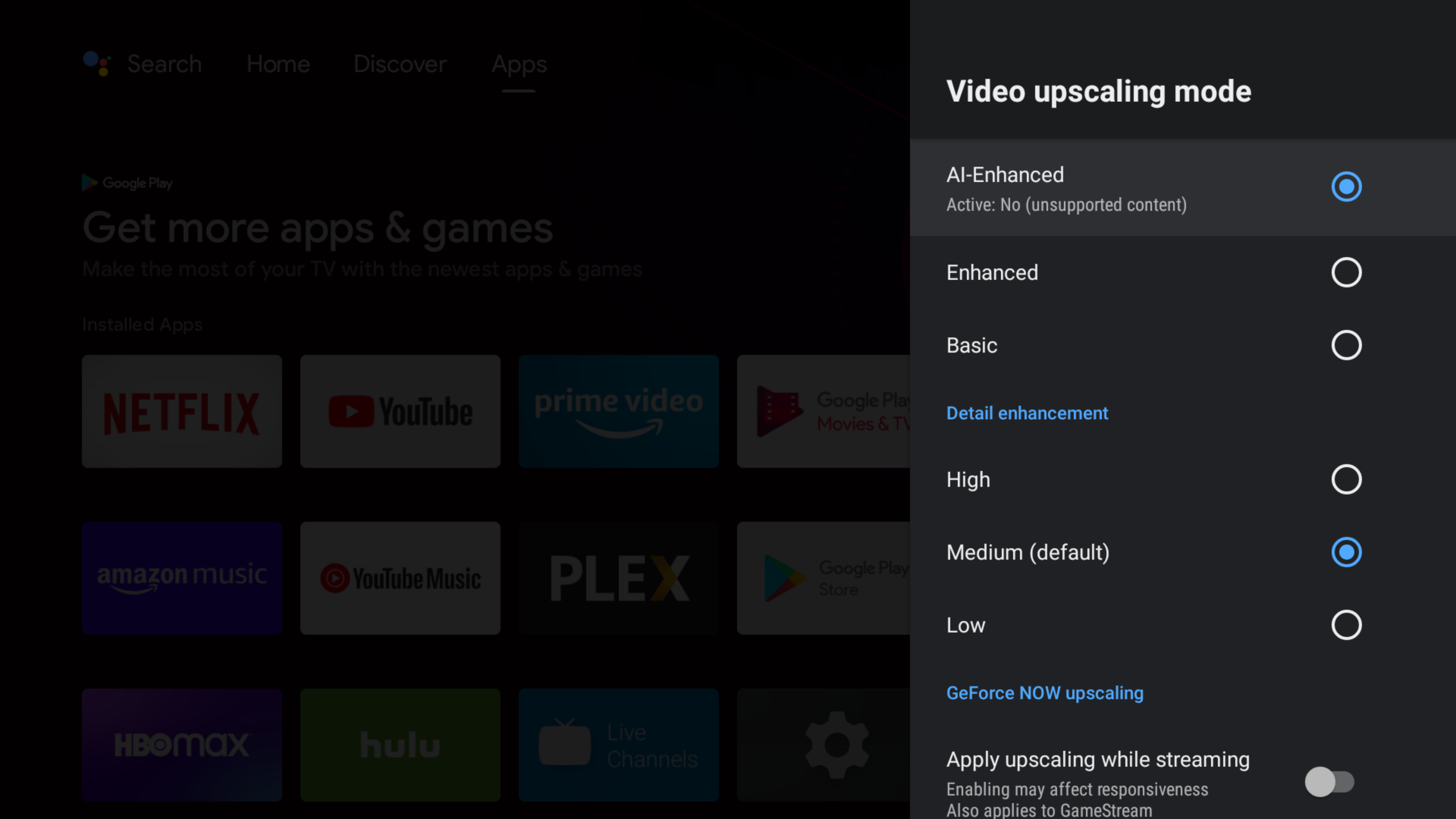The image depicts a screen perceived from either a laptop or smart TV, showing a partially grayed-out background with visible menu options. At the center, a line of text reads "Get More Apps and Games" in white, under which several app icons are lined up. Among the recognizable app icons are Netflix, YouTube, Prime Video, Amazon, HBO Max, Plex, Hulu, and a gear icon representing the options menu. Additionally, there is an unclear icon that resembles Google Chrome or a similar app.

On the left side of the screen, the options menu is open. It highlights a setting for video upscaling mode, offering various choices: AI Enhanced, Active, No Unsupported Content, Enhanced, Basic, Detail Enhancement, High, Medium, and Low. The upscaling feature, known as GoForce Now, is designed to apply upscaling while streaming content.